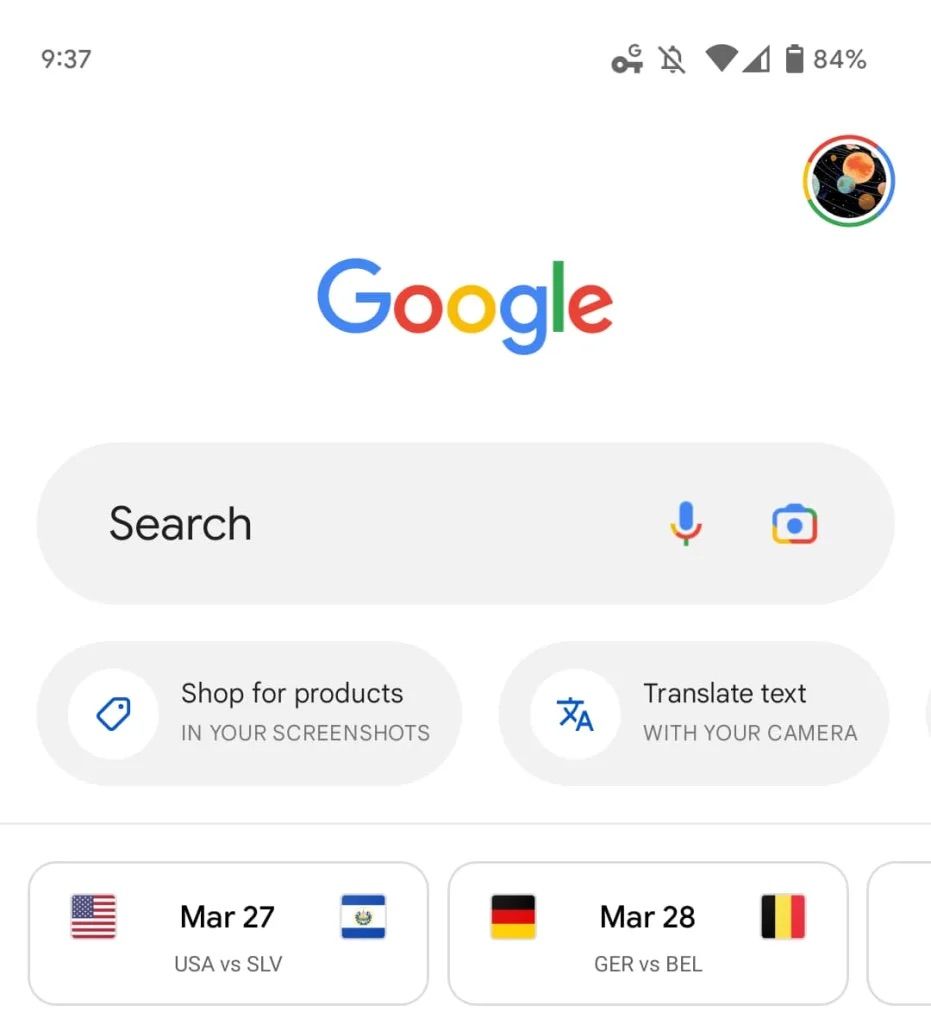The image depicts a detailed smartphone screen, capturing various icons and notifications. In the upper right corner, a cell phone battery icon indicates an 84% charge. Adjacent to it, a bell icon with a diagonal slash signifies that notifications are muted. On the left, the time is displayed as 9:37.

Beneath the battery icon, a circular icon featuring a black background and small, circle-shaped orange and blue planets is visible. Below this, the word "Google" is prominently displayed in capital letters (G-O-O-G-L-E), accompanied by a large search bar with rounded ends containing the text "search." To the right of the search bar, there's a blue microphone icon and a multi-colored box representing Google colors: blue, red, yellow, and green.

On the left side, an icon depicts a circle with a shopping tag inside it, alongside the text "shop for products." Below it, "in your screenshots" is mentioned. To the right, another white circle features an "A" with a line above it and an "X" below the line, with the caption "translate text with your camera."

In the bottom left corner, a rectangle displays an American flag and the date March 27th, followed by "USA vs. SLV." Next to it, a square icon features the black, red, and yellow colors of the German flag, the date March 28th, and "GER vs. BEL."